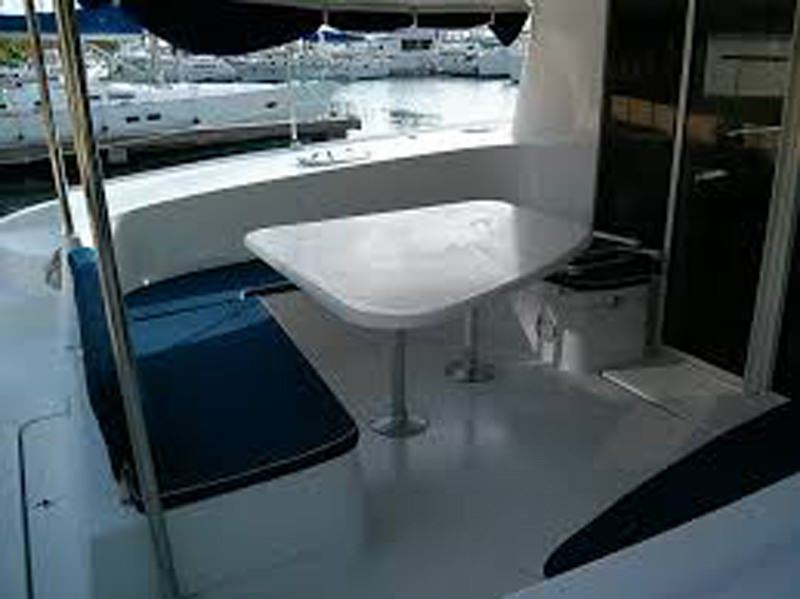This outdoor photograph, likely taken during the day from the back of a boat, captures a seating and dining area with blue cushioned benches and a small rectangular table positioned between them. Above the seating area hangs a shade or awning, providing partial cover. To the right of the table is a dark doorway leading into the interior of the boat. The boat itself sports a predominantly white color scheme, matching other boats docked nearby. The scene extends to a marina or harbor setting with calm waters and stationary white boats, some with small windows visible. Slight greenery can be spotted in the top left corner of the image. However, the photograph is heavily compressed with significant JPEG artifacting and blurriness, rendering fine details indistinguishable.